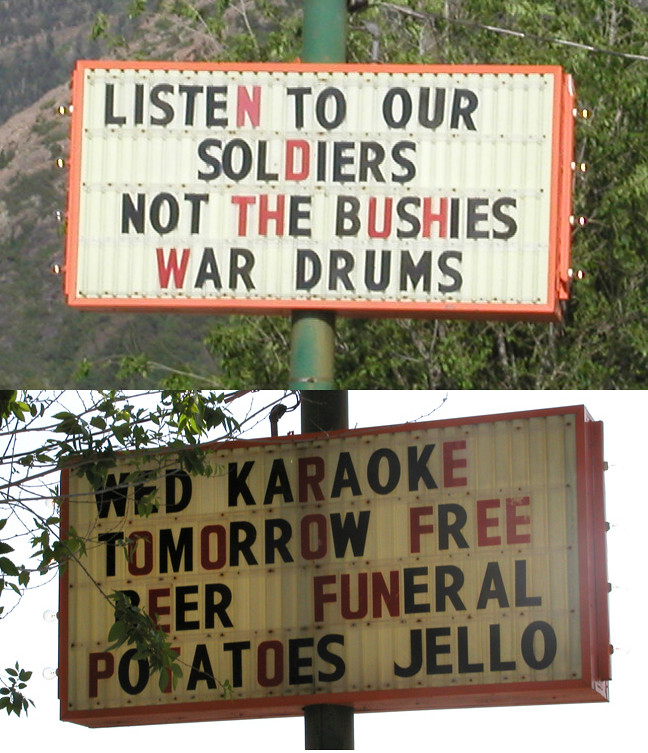The image comprises two divided sections, each featuring a sign mounted on a green pole. The top section displays a white sign with a red border, constructed of small lettered panels. It reads: "LISTEN (with 'N' in red and the rest in black) TO (in black) OUR (in black) SOLDIERS (with 'SOL' in black and 'DIERS' in black) NOT (in black) THE (with 'TH' in red and 'E' in black) BUSHIES (in black) WAR (in black) DRUMS (in black)." The background presents an array of trees. 

The bottom section shows a similar sign on the same green pole. Unlike the top section, the background here includes only one tree situated in front of the sign. This sign contains an unusual message spelled out in a continuous string of black letters: "WEDKARAOKETOMORROWFREEBEERFUNERALPOTATOESJELLO."